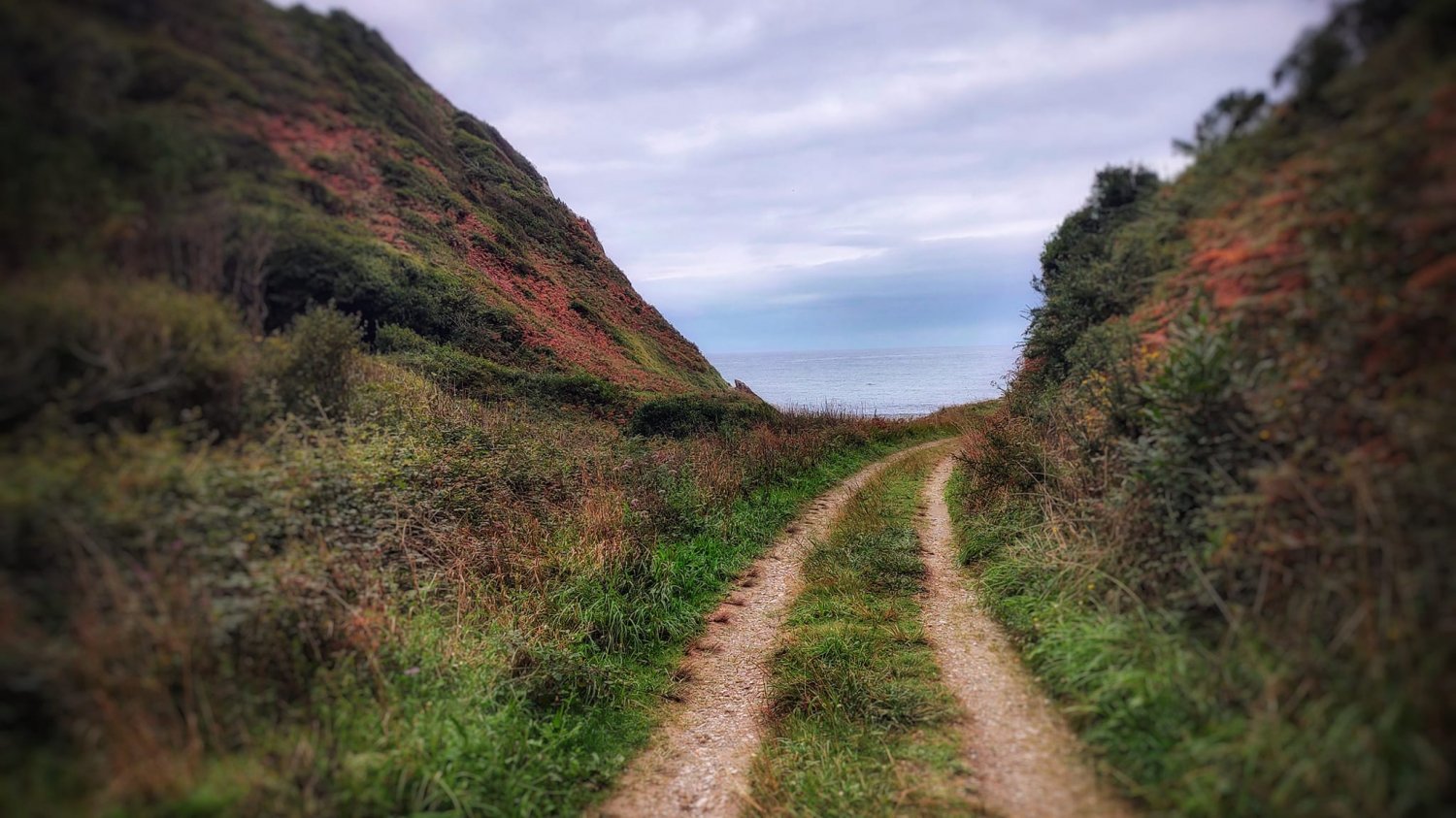In this image, a dirt trail winds between two steep hills, which rise prominently on either side. The hills are a patchwork of muted browns, beiges, and greens, dotted with short vegetation, and the occasional reddish flowers, giving them a slightly desolate appearance. The trail itself consists of two parallel tire tracks separated by a strip of grass that has grown tall and overgrown, indicating infrequent use. Along the edges of the trail, the grass is lush and green, contrasting with the drier vegetation on the hills. As the trail curves off to the right in the distance, the horizon reveals a glimpse of the ocean, its light gray-blue waters blending seamlessly into a sky filled with flat, white clouds. The overall scene is serene yet slightly rugged, capturing the quiet beauty of an untamed landscape.